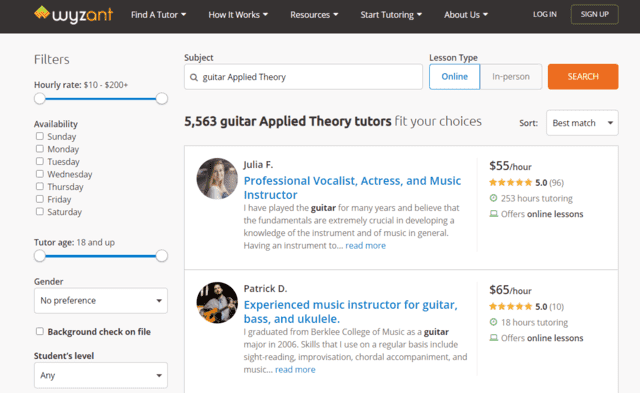The image showcases a webpage on the Wyzant website, which specializes in tutoring services. The page prominently features sections such as "Find a Tutor," "How It Works," and "Resources." The focus of the search appears to be on finding a tutor for guitar applied theory. Two tutor options are highlighted: 

1. **Julia** - A professional vocalist, actress, and music instructor, offering her services at a rate of $65 per hour.
2. **Patrick D** - An experienced music instructor who specializes in guitar, bass, and ukulele, available for $55 per hour.

The layout suggests a user-friendly interface, guiding the user through the process of selecting a suitable tutor based on their specific needs and budget.